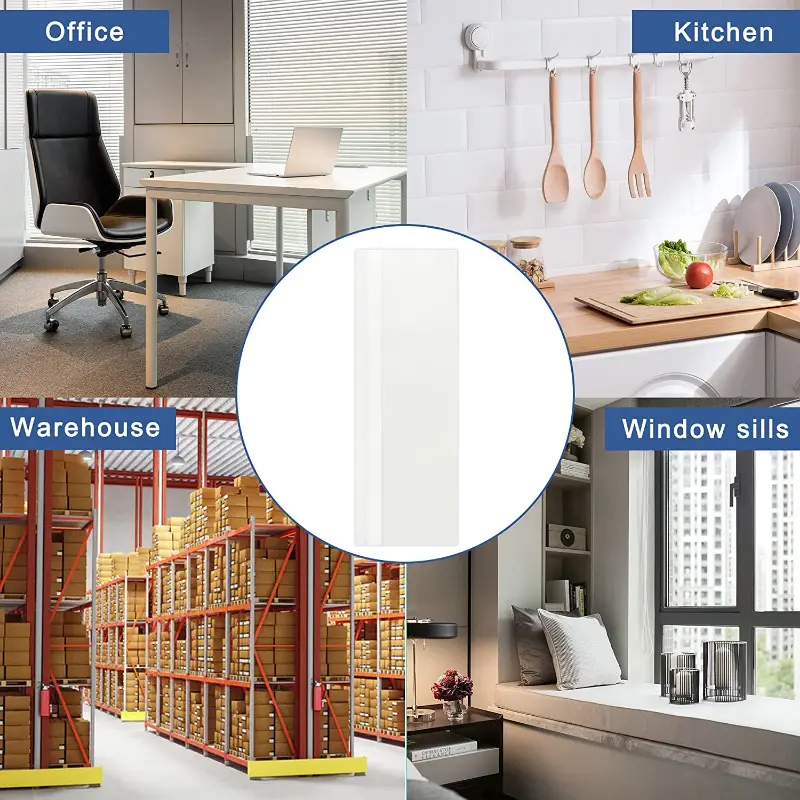The image is a digitally created composition featuring four distinct sections arranged in a 2x2 grid, with each section clearly labeled in blue rectangles with white text. In the center of the grid, a white circle with a light gray rectangular detail combines all four sections. 

The top-left section, labeled "Office," shows a modern workspace with a black office chair on wheels in front of a white desk that holds an open laptop. Behind the desk is a white cabinet, and the room features a tan carpet.

The top-right section, labeled "Kitchen," depicts a wooden countertop beneath a white, brick-style backsplash. Hanging on the wall above the counter are wooden utensils, including two spoons and a fork. The counter also displays a cutting board with a tomato and some lettuce, as well as a few plates.

The bottom-left section, labeled "Warehouse," presents a storage area with sturdy metal shelves on a gray cement floor. The shelves are filled with various small wooden and cardboard boxes.

The bottom-right section, labeled "Window Sills," showcases a window sill adorned with a couple of pillows, offering a view of a distant skyscraper.